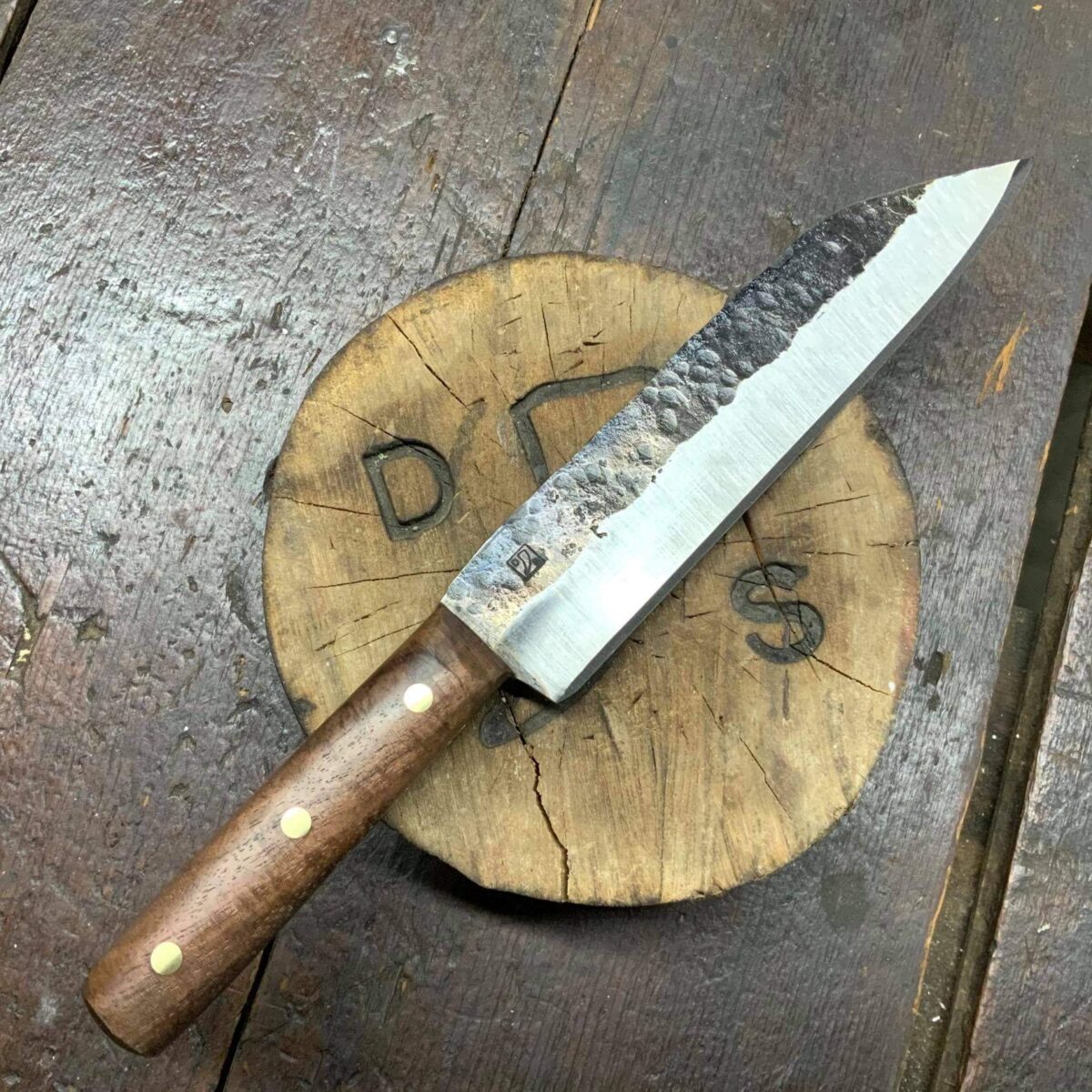The photograph showcases a weathered, dark wooden table with fine lines, dings, and marks. Positioned on the table is a light beige-brown coaster adorned with partially visible letters "D" and "S," obscured by a knife resting on it. The knife features a brown handle with gold rivets and a stainless steel blade that appears used, given the debris on its upper edge. Its shape reminds one of a butcher's knife, though it is smaller. The overall composition highlights the rustic and utilitarian character of these objects in a detailed and evocative way.